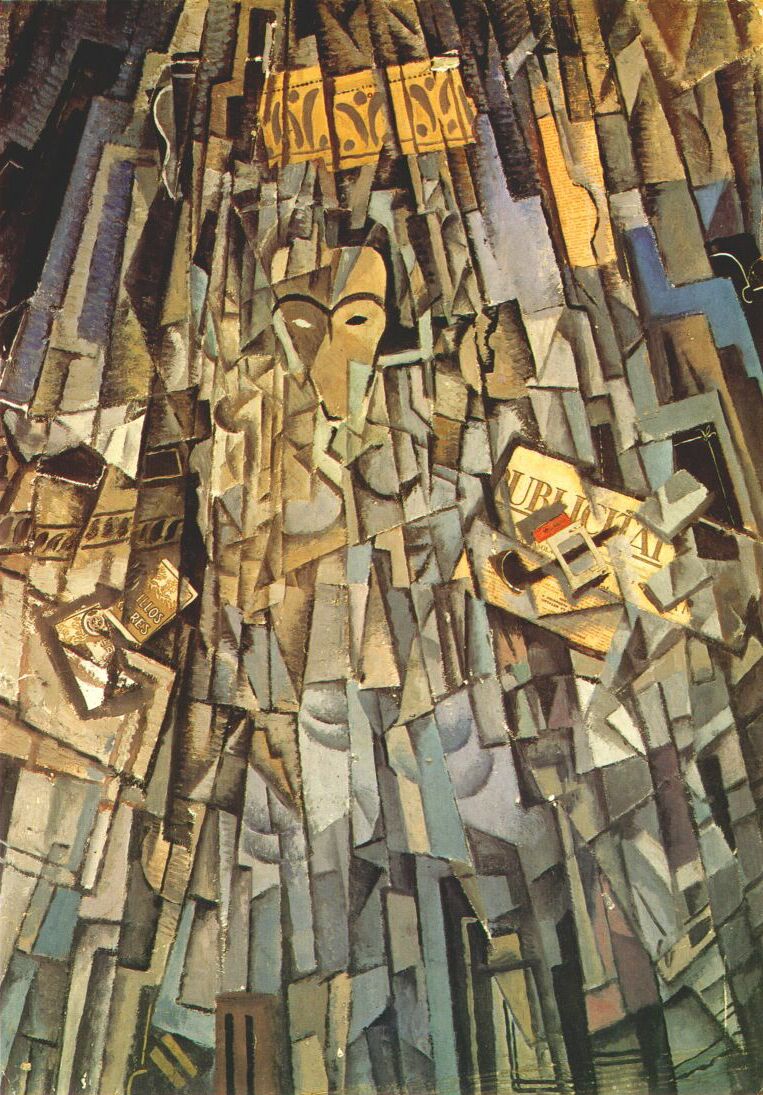The image is a vertical, abstract collage or painting, largely composed of geometrical shapes and shards, reminiscent of a deconstructed and reassembled stained glass window. It prominently features various shades of brown, along with accents of blue, gray, black, yellow, tan, beige, and gold. The central figure appears to be a fragmented, almost animated, human-like shape, vaguely resembling a distorted face with lines representing a nose, eyes (one light and one dark), and curved lines that could symbolize brows. The human figure is set within a chaotic mosaic that evokes the shattered and reassembled style of a Picasso artwork, contributing to an overall modernist aesthetic. Scattered throughout the composition, there are indistinct bits of text and possibly advertisements, including what looks like a pack of cigarettes near the right side. The geometrical elements dominate the entire painting except for the top left corner, reinforcing the abstract nature of the piece.